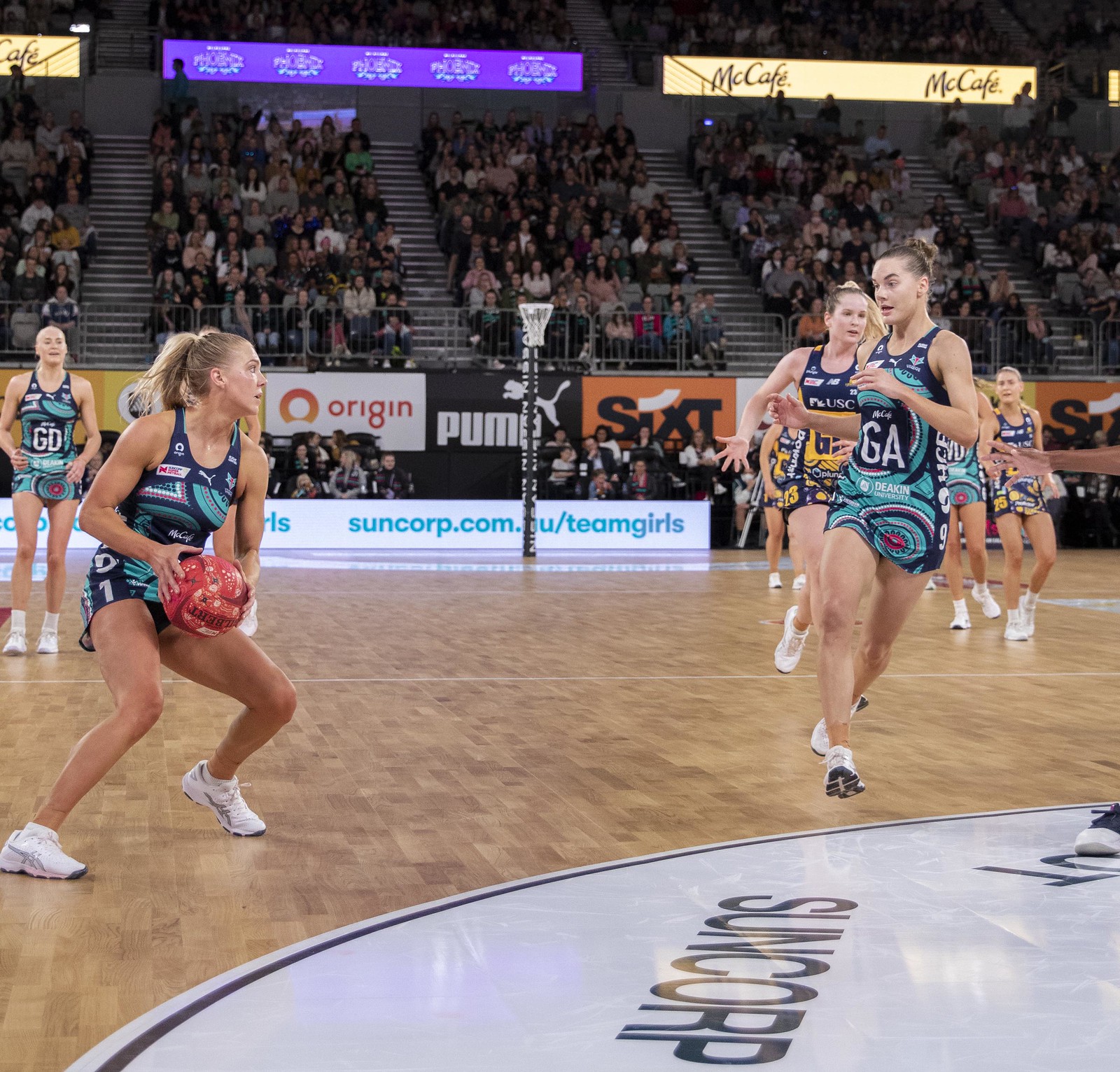In the image, there is a vibrant indoor scene capturing a girl’s basketball game. The polished, light brown wooden floor is scattered with patches of paint, indicating a well-used court. Central to the image are the players, with one girl clearly in possession of the ball. The players are split into two teams; one team is clad in green and dark blue uniforms, while the opposing team wears yellow and blue. Adding further splashes of color, one girl’s outfit features white, pink, and blue, complemented by green and white shoes.

The audience is seen in the background, filling the stands and intently watching the game. Several advertisements are visible, notably "Sun Corp" on the court itself in a mix of white, red, and dark blue lettering, and "McCafe" prominently displayed in the background. Another advertisement reads "Origin Puma 6th," although part of it is obscured by a pole. The setting is bustling with activity, suggesting it is during an intense and active game. The image captures the lively atmosphere of a competitive basketball match inside a spacious, well-lit stadium.